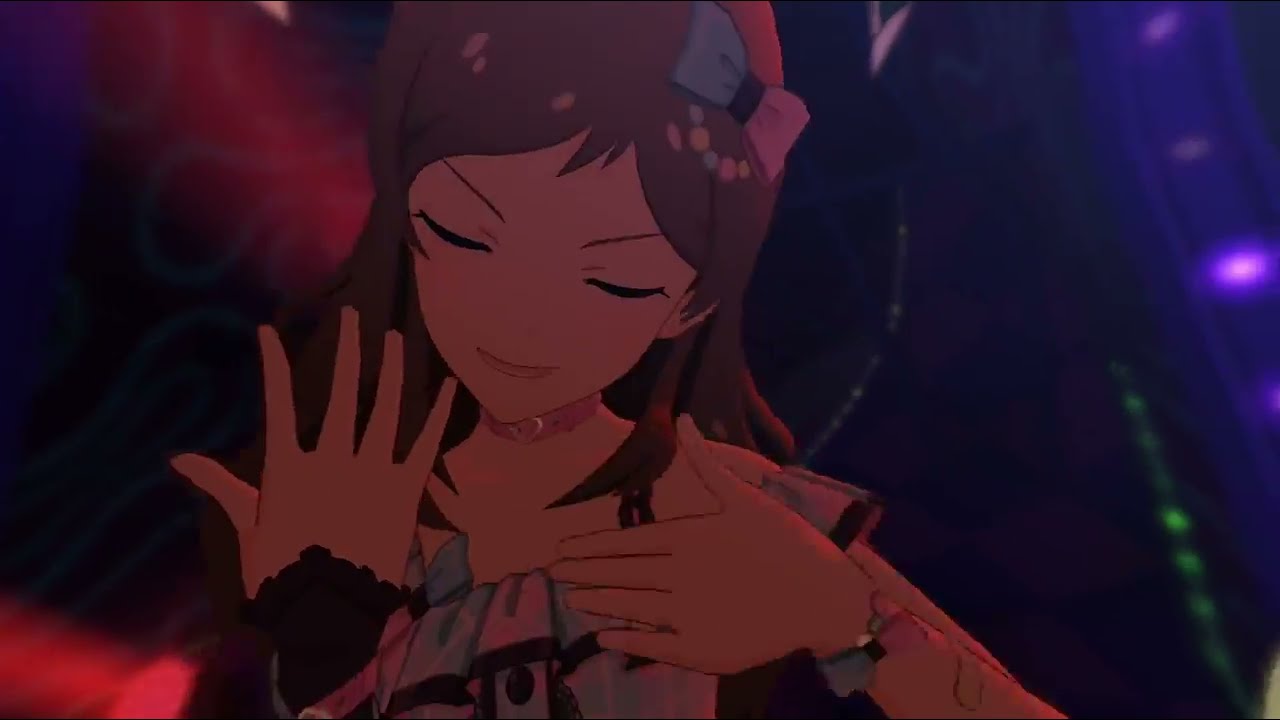The image features a detailed and intricate still of a brown-haired animated girl from an anime. She has long, pointy hair cascading both in front and behind her, adorned with a bow that is gray and pink on one side, and blue and pink on the other. Her eyes are closed, and her thin eyebrows accentuate her delicate and pointy chin. She also has light skin and thin lips. The girl is wearing a pink choker around her neck and a frilly, off-the-shoulder top that is white, with ruffles lining her arms. Her left hand is raised with fingers pointing up, while her right hand rests near her chest, adorned with a black lacy wristband. In her hair, there are additional beads adding to her ornate appearance. The background is an abstract mix of dark tones with colorful highlights, featuring purple, green, blue, and red hues, which add a sense of vibrancy and dynamics to the scene. On the right, there's a notable purple arch with lights, enhancing the ethereal atmosphere.